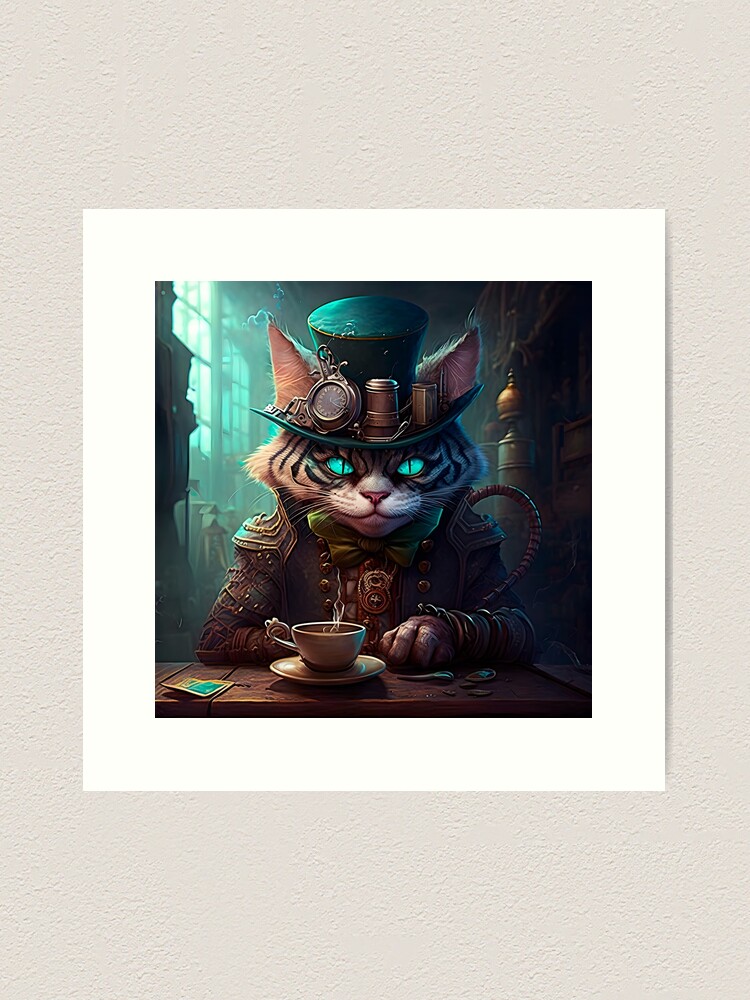The digital artwork displayed on a light gray, textured wall as a square print with a thick white border, showcases a detailed 3D illustration of a steampunk-styled cat. The cat, with its striking teal eyes and striped gray fur, sits upright at a wooden table. It wears a black top hat adorned with a clock and various steampunk elements, including implements and gauges. The cat is dressed in a shoulder-padded, steampunk-inspired jacket made of leather and metal, complete with a gauntlet on its right paw. In front of the cat is a steaming ceramic cup and saucer, possibly containing coffee or tea. To the left of the table, there are cards, and to the right, a collection of other items. A window in the background lets in teal light, enhancing the surreal and imaginative ambiance of the scene.